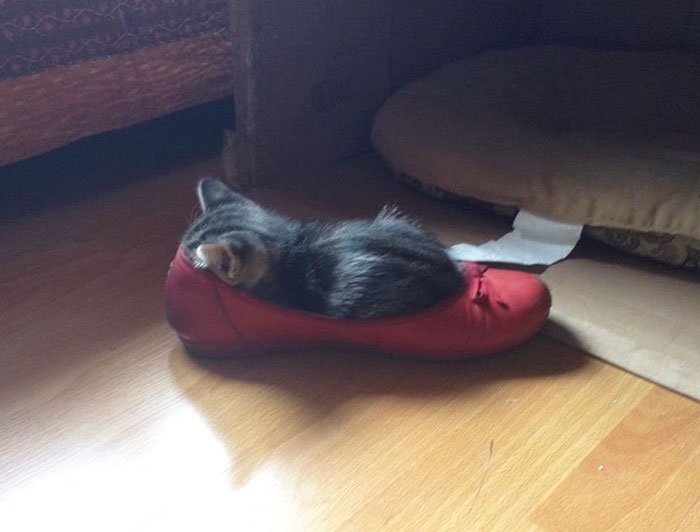This photograph, though a bit grainy and slightly blurry, captures an endearing scene of a black and white kitten nestled inside a red women's flat shoe, which features a delicate bow on its toe. The shoe is positioned on a wooden floor, pointing to the right. The kitten, too small to fit comfortably, has its head tucked into the heel part of the shoe, with only its ears visible, and its body spilling out towards the toe. In the background, to the upper right of the image, there is a beige cat bed with a white tag, situated inside a cardboard box. Additionally, in the upper left corner, a piece of material, possibly a bed sheet, is visible. The photo's overall dark tones provide a cozy ambiance, further highlighting the kitten's charming choice of an unconventional resting spot.